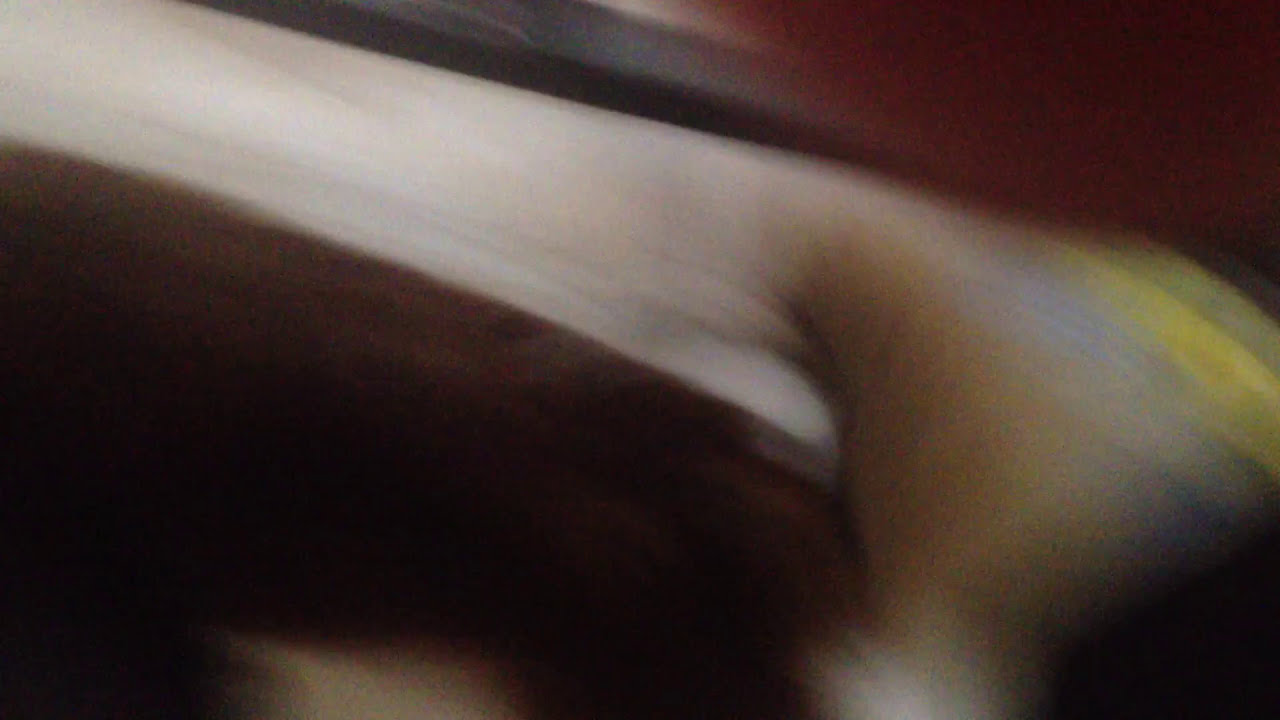The image is a dynamic and abstract photograph capturing what seems like a swirling motion, possibly of someone kneading or spinning dough. The composition features a prominent white streak or blur starting from the top left, extending towards the center, where it transitions into various colors. The streak is white and light at the start, gradually darkening into brown as it moves rightward, with an amber spray paint effect in the upper right corner. Towards the center, the streak gains a yellow hue on the right. The lower left corner of the photograph is predominantly dark, with shades of black and a small gray blotch slightly right of the corner. Overall, the photograph has a grainy texture, adding to the sense of motion and obscuring finer details, making the central white, dough-like structure, and the possible outline of a hand moving, appear fluid and indistinct. The background features deep reds in the upper right and darker hues in the lower sections, contributing to the swirling, dynamic effect of the image.